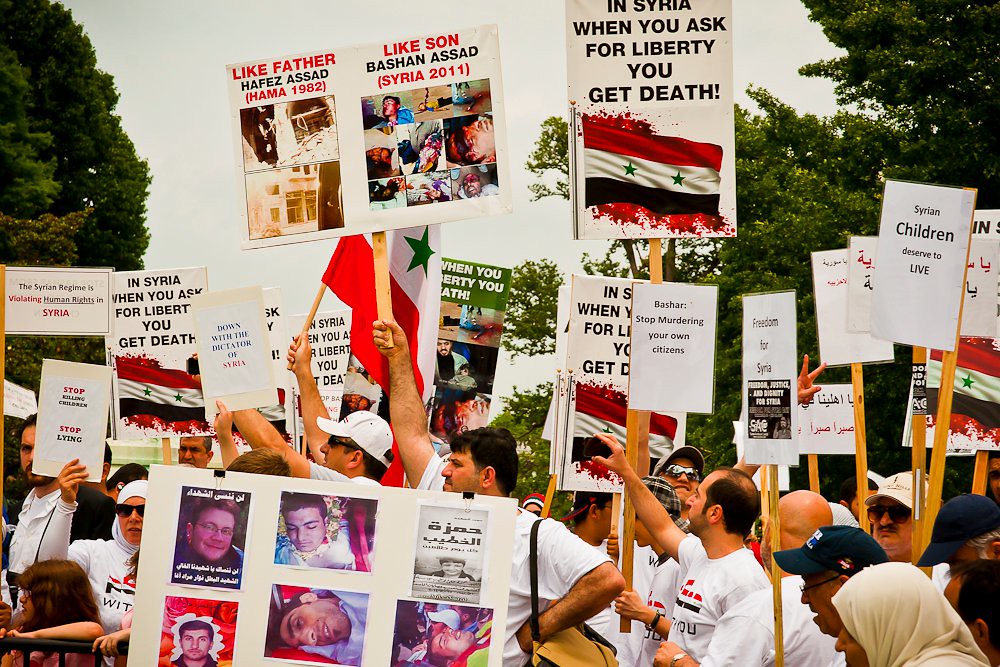This daytime photograph captures an outdoor protest, presumably against the Syrian conflict, with approximately 20 to 30 worried-looking protesters in the frame, many of whom are donning white T-shirts. Among the protesters are women wearing headdresses. The backdrop features several trees and a white-hued sky. The protesters are holding up white placards mounted on wooden sticks, prominently featuring messages and images. One notable sign reads, "In Syria, when you ask for liberty, you get death," accompanied by a Syrian flag with red, white, and black stripes and two green stars. Another sign powerfully declares, "Like father, Hafez Assad, Hama, 1982. Like son, Bashan Assad, Syria, 2011," with a collage of graphic, heart-wrenching images of casualties. Additional signs passionately proclaim, "Syrian children deserve to live," "Stop murdering your own citizens," and "Freedom for Syria." The protesters are directing their attention off to the left side of the photo, away from the photographer.